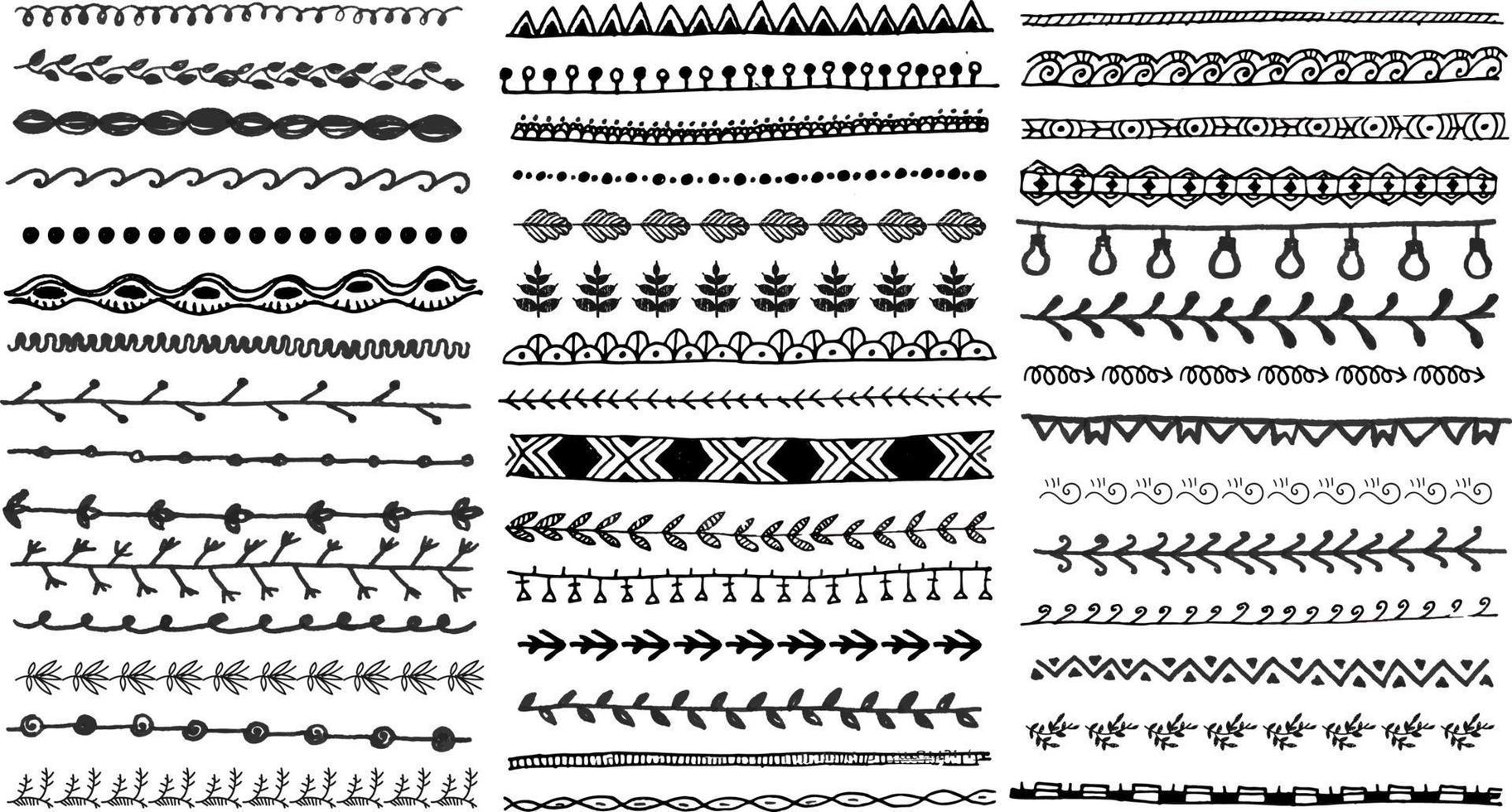In this intricate black-and-white image, we see three rows filled with various patterns and designs on a white background, resembling detailed illustrations on pieces of cloth. Starting from the left-hand side, the patterns descend methodically, beginning with squiggly lines and followed by what look like vining leaves, circular loops, and waves. This row also includes dots, mountain-like shapes, a straight line with small perpendicular lines, and another with dots. Further down, we see more floral and leafy motifs, culminating in complex, interconnected designs reminiscent of octopuses, puka shell necklaces, and seaweed.

The central row features a mix of similar patterns but with a distinct thick line adorned with white X's that stands out prominently. This row includes pyramids, vining leaves, various symbolic lines, and flowing waves. Many of the designs are connected, with an array of nature-inspired motifs like evergreen trees, flowers, and intricate geometric shapes, adding a textured richness to the sequence.

The rightmost row showcases increasingly complex symbols, including hanging lights, more waves, and leaf patterns. It also features an array of uniquely adorned lines—from those with white squares to ones resembling Native American necklaces and fern leaves. The detailed continuity of designs on this side closes with sequences of chain-like necklaces and wavy, interconnected forms, creating a tapestry of diverse patterns across all three rows.